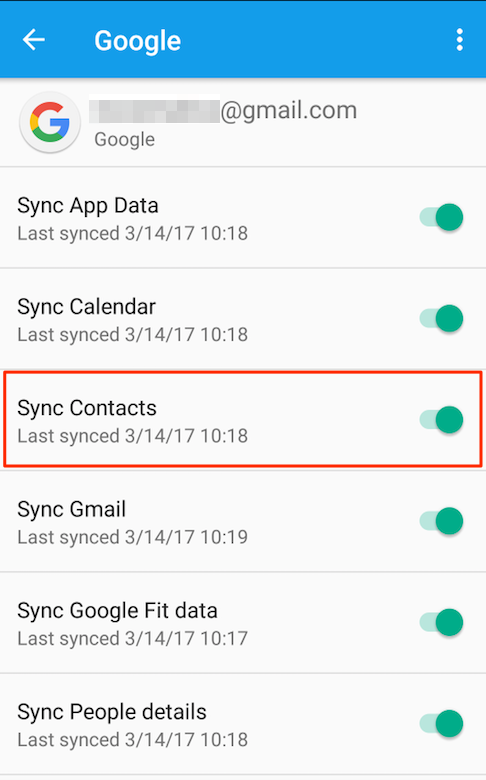The image showcases a Google synchronization settings page. At the top of the page, a blue bar stretches horizontally from left to right. On the left side of this bar is a back arrow, while the right side features three vertically aligned dots. Beneath the blue bar, you can see the Google logo with its distinctive red, blue, yellow, and green colors.

Underneath the logo, there's a grayed-out email address ending with "@gmail.com," partially blurred for privacy. Below the email address, the word "Google" appears in gray text, and the settings categories follow.

The first category listed is "Sync app data," with a note indicating that the data was last synchronized on March 14, 2017, at 10:18 AM. A slider next to this category allows the user to enable or disable synchronization.

The second category is "Sync calendar," which was last synced on the same date and time. 

The third category, "Sync contacts," is highlighted with a red outline and also shows the same last synchronization date and time.

Next is the "Sync Gmail" category, last synchronized on March 14, 2017, at 10:19 AM.

Following that is the "Sync Google Fit data" category, last synced a minute earlier at 10:17 AM.

Finally, the last category is "Sync people details," with its last synchronization timestamp also being March 14, 2017, at 10:18 AM.

All these synchronization options are accompanied by green sliders that can be toggled on or off.